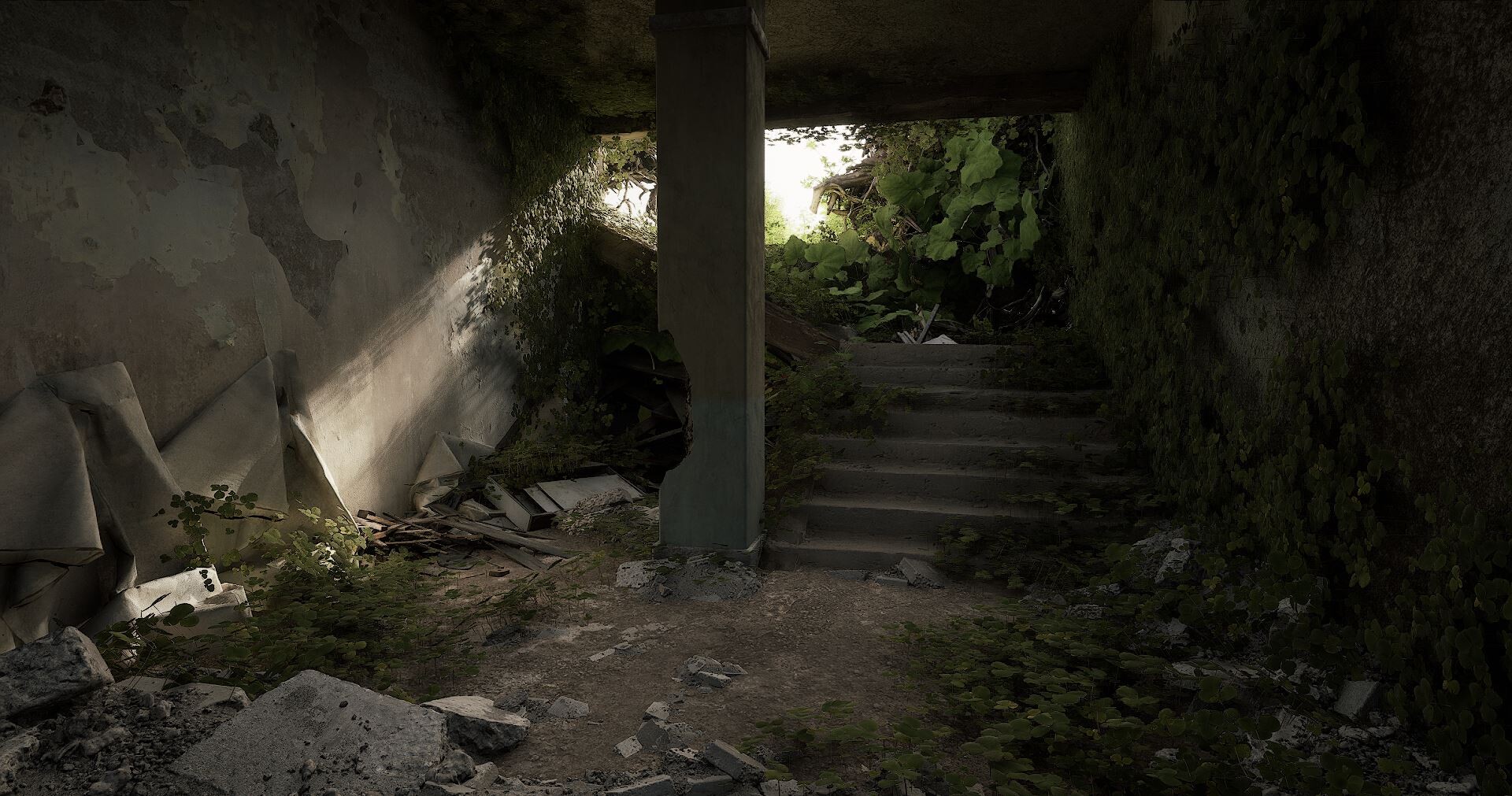This photo captures a dilapidated, underground space that appears to be the remnants of an abandoned shelter, basement, or old overpass. The lower area is dark and scattered with broken pavement and rocks. A crumbling pillar with a noticeable hole supports an upper level from which sunshine spills down, illuminating part of the basement. There are dull, purposely constructed cement stairs leading from the lower level up to the overgrown upper level, where green leaves and trees are visible. The decaying walls are peeling with plaster, covered in ivy, and patches of moss. The image gives a haunting sense of abandonment, possibly from a past demolition, house fire, or natural decay, with rubbish and vegetation scattered throughout. The perspective is taken from human eye level, facing the stairs, emphasizing the stark transition from the shadowy underground to the sunlight above.